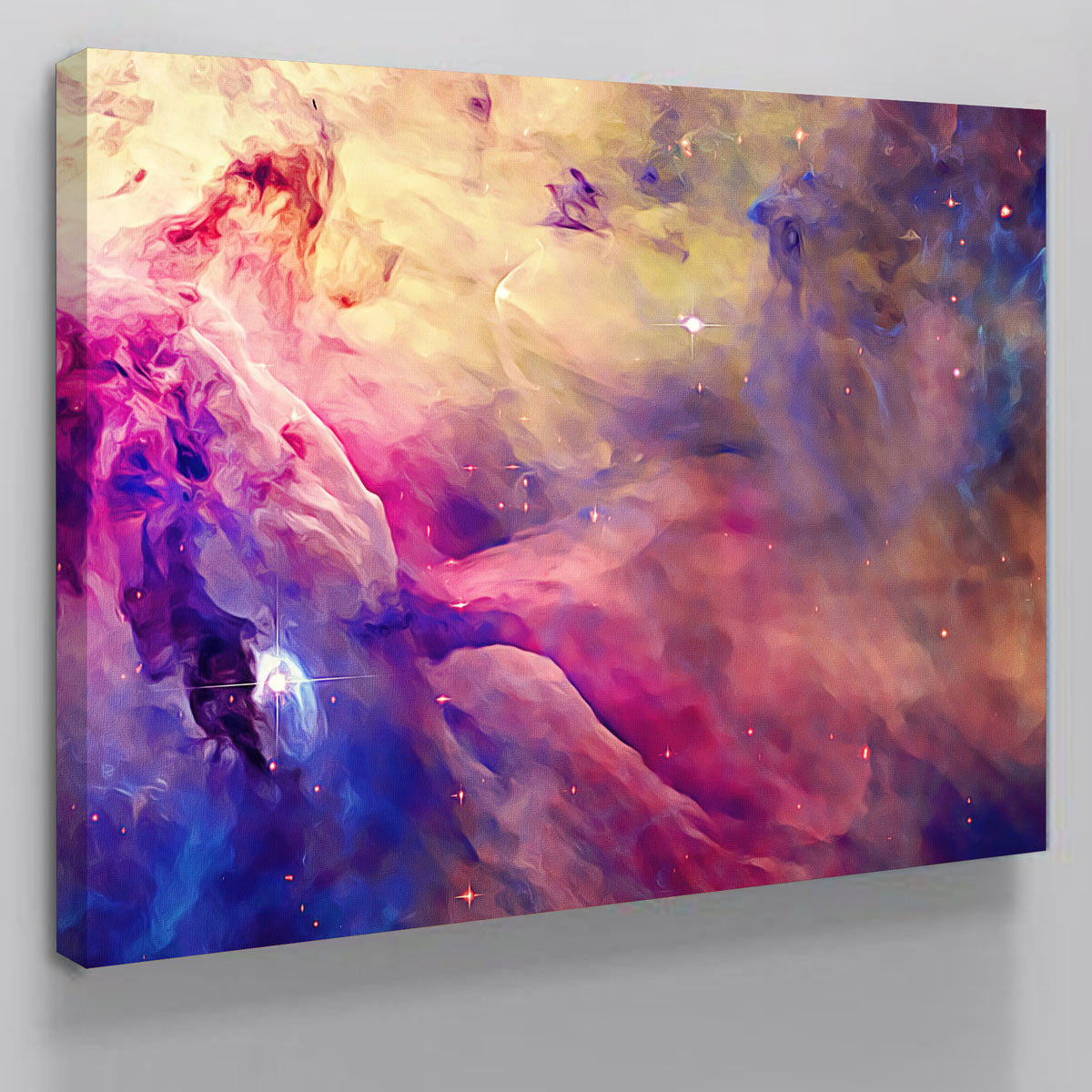This image captures an abstract, large rectangular canvas painting that hangs on a light gray wall. The painting vividly depicts a dreamy, night-time sky scene resembling a galaxy, with artfully blended, smoky areas of various colors. The top section of the painting exudes soft hues of yellows and creams, while the upper left and right corners have infused purples with delicate cloud effects. Descending through the canvas, vibrant shades of pinks and reds transit into the bottom left corner, bursting into bright purples and blues. Scattered throughout the painting are numerous bright dots representing stars. Notably, there is a striking white circle reminiscent of a radiant star near the center-right, and another luminous white star embedded in a wispy white cloud at the top. The painting's edges are wrapped around the sides, enhancing its immersive effect, and it predominantly fills the image frame, emphasizing its grandeur and allure.